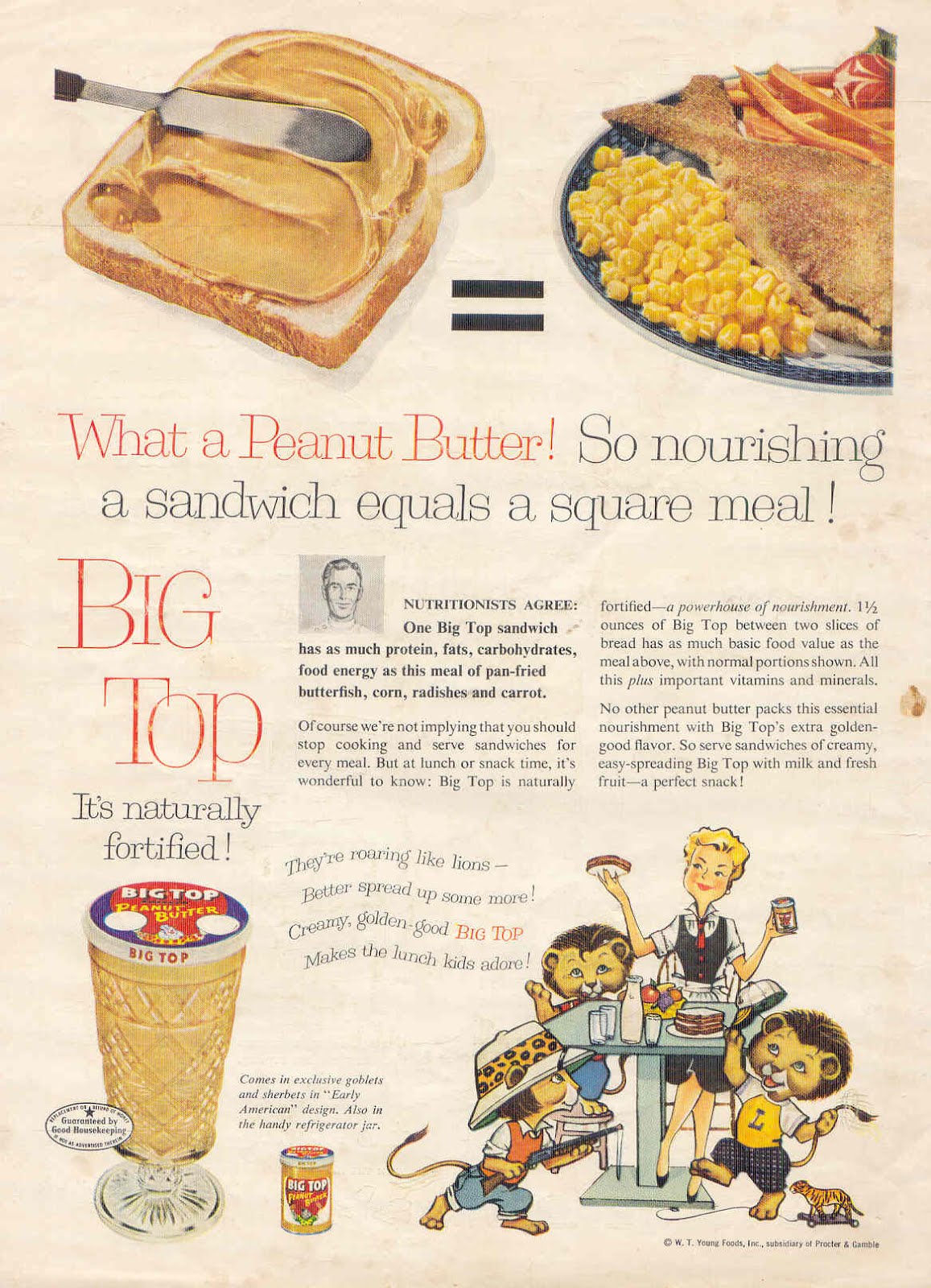The vintage-style illustration appears to come from a 1950s or 1960s magazine advertisement for Big Top Peanut Butter. At the top of the advertisement, a slice of white bread with peanut butter being spread by a silver knife is depicted. Next to it, an equals sign links this image to a plate of nutritious food featuring fried fish, corn, carrots, and possibly radishes, implying the peanut butter sandwich matches the meal's nutritional value. The tagline reads, "What a peanut butter! So nourishing. A sandwich equals a square meal!" 

The ad emphasizes that Big Top peanut butter is naturally fortified, highlighting its nutritional equivalence to a well-balanced meal with the statement: "Nutritionists agree one Big Top sandwich has as much protein, fats, carbohydrates, and food energy as this meal of pan-fried butterfish, corn, radishes, and carrots." The text further assures that while the brand is not suggesting a complete replacement of meals with sandwiches, Big Top provides a nutritive and convenient option for lunch or snacks.

In the detailed illustrations below, the advertisement shows a mother holding a plate and a jar of Big Top peanut butter, serving sandwiches to her children, who are illustrated as lion cubs dressed in human clothing, symbolizing their energetic and playful nature. Accompanying the family scene is a picture of the Big Top peanut butter jar, described as coming in exclusive goblets and sherberts with an early American design, and also available in a practical refrigerator jar.

The ad concludes by promoting Big Top’s creamy and easy-spreading texture: "Serve sandwiches of creamy, easy spreading Big Top with milk and fresh fruit—a perfect snack." Overall, Big Top Peanut Butter is presented as a powerhouse of nourishment, packed with essential vitamins and minerals, bearing the heroic endorsement: "No other peanut butter packs this essential nourishment with Big Top's extra golden good flavor."